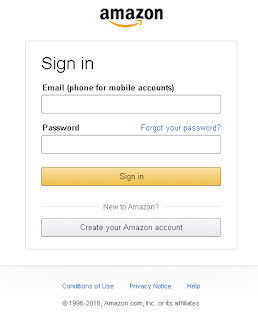A closely cropped screenshot of the Amazon sign-in page on a mobile device features a clean, white background. At the top center, the distinctive Amazon logo is prominently displayed. Below the logo, a sign-in form is enclosed within a thin gray border. Exuding a minimalist design, the form is divided into several sections. 

At the top left of the form, "Sign-In" is written in black. Directly below, fields for "Email" (with an indication that a phone number can be used for mobile accounts in parentheses) and "Password" are ready for input. Adjacent to the Password field, a "Forgot your password?" link is presented in blue text for users who need assistance.

An input field for the password appears immediately below these sections, followed by a conspicuous, orange "Sign-In" button, occupying a significant portion of the screen for easy access.

Centered at the bottom of the sign-in form, a prompt for new users appears: "New to Amazon?" in light gray, followed by "Create your Amazon account" which is also in gray but styled as a clickable button for account creation.

Beneath the sign-in form, three essential hyperlinks— "Conditions of Use," "Privacy Notice," and "Help"— are lined up at the center. At the very bottom of the screen, a footer note reads, "© [current year] amazon.com, Inc. or its affiliates," underscoring the company's policies and trademarks.